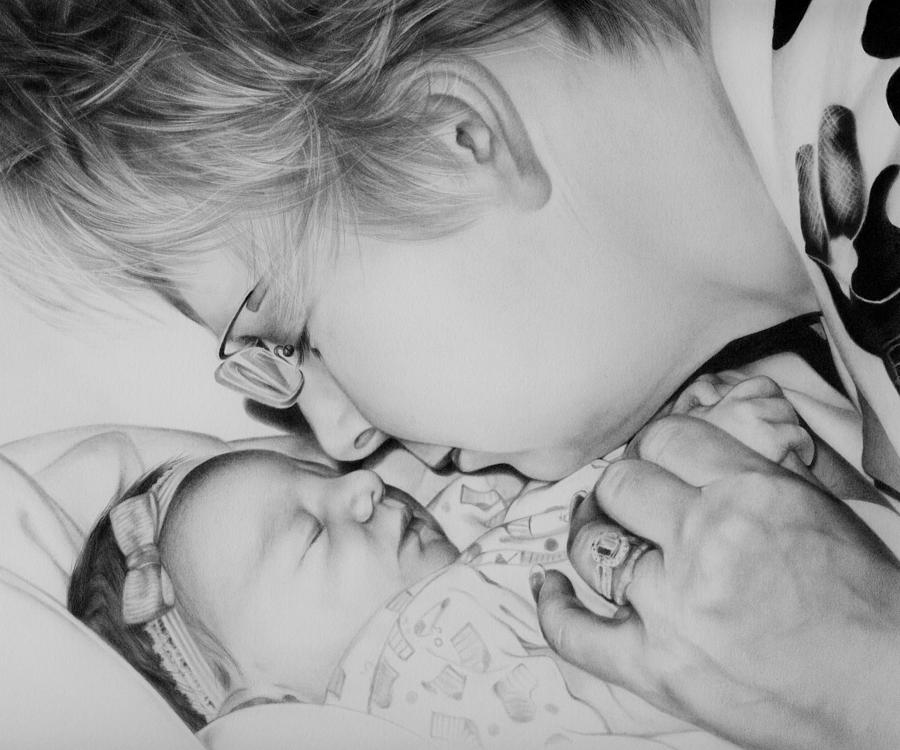This is a black-and-white photographic image set indoors, capturing a touching moment between a woman and a newborn baby. The woman, who appears to be white with short blonde hair, is wearing glasses and a floral print dress. Her head and shoulders are visible as she lovingly leans over to kiss the sleeping baby, who is adorned with a headband and wrapped in a blanket. The image highlights the close bond between the two, as the woman's nose gently touches the baby's nose. The woman is also wearing a wide band ring on her left ring finger, adding a subtle detail to her appearance. The composition of the photograph, marked by delicate shadings, brings out the intimate and heartwarming essence of the scene.